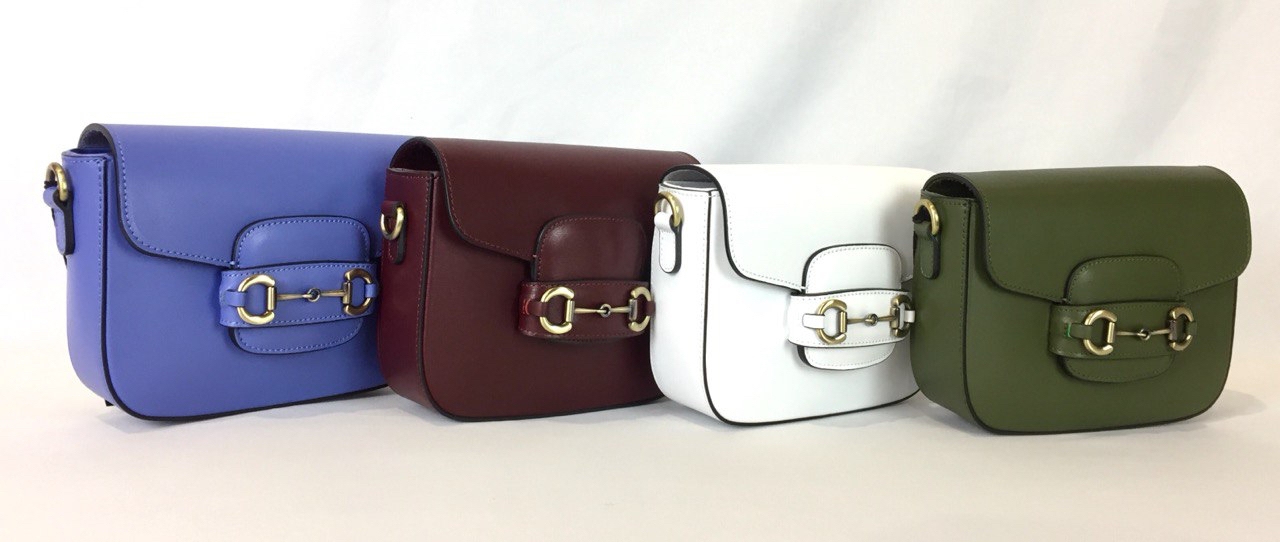This photograph features a set of four handbags, each identical in design but varying in color, arranged to partially overlap diagonally against a white background. The bags all feature gold accents, specifically rings around the straps and front clasps. From left to right, the colors are blue, maroon, white, and olive green. The consistent gold detailing and matching design suggest a coordinated collection, indicative of a professional photo shoot likely aimed at advertising a new brand release.